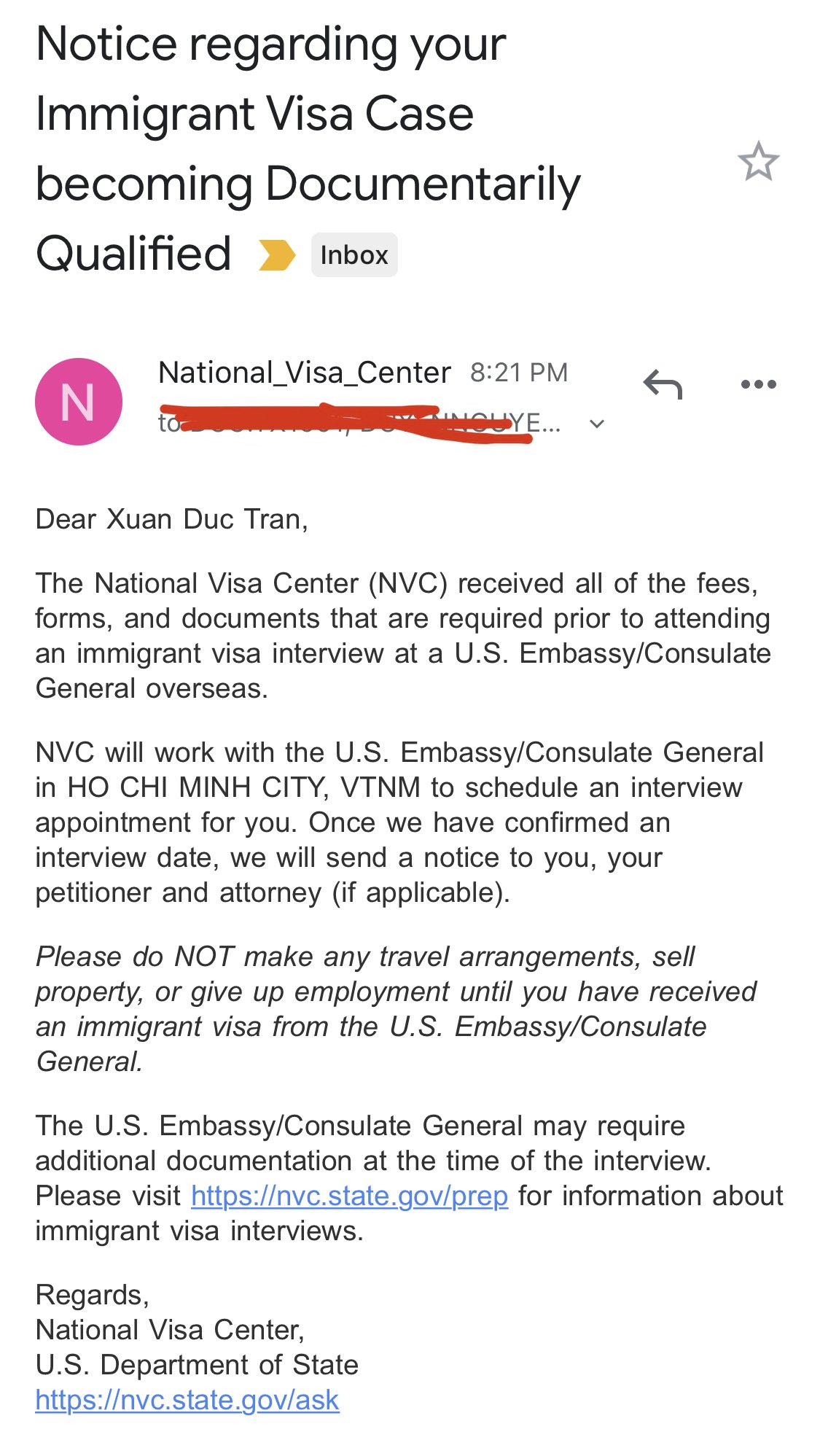Notice Regarding Your Immigrant Visa Case

The National Visa Center (NVC) has received all of the required fees, forms, and documents for your interview at the U.S. Embassy or Consulate General overseas. Specifically, the NVC will coordinate with the U.S. Consulate General in Ho Chi Minh City, Vietnam, to schedule your interview appointment.

Once a date has been confirmed, a notification will be sent to you, your petitioner, and your attorney (if applicable). It is important that you do not make any travel arrangements, sell property, or resign from employment until you have received your immigrant visa from the U.S. Consulate General. 

Please be aware that additional documentation may be required at the time of your interview. For more information about immigrant visa interviews, please visit the official website provided in the correspondence.

Regards,
National Visa Center
U.S. Department of State